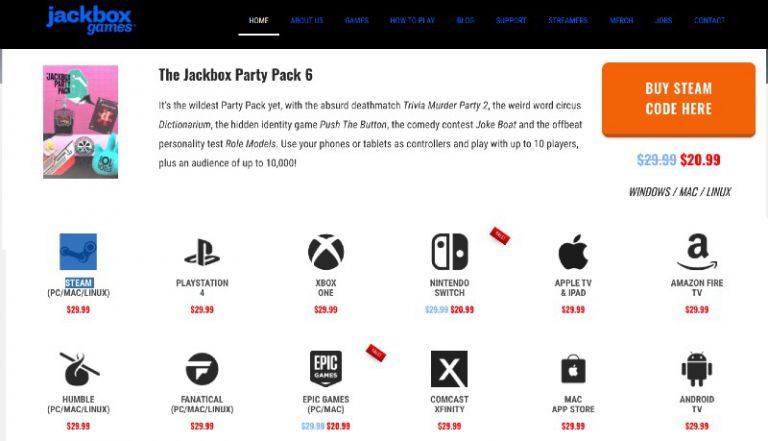**Detailed Caption for the Screenshot:**

This image is a detailed screenshot of a website’s store page showcasing a digital product. The header of the website is black, prominently displaying a blue logo in the top left corner that reads "Jackbox Games." The word “Jackbox” is positioned above and “Games,” in italics, is centered beneath "KBOX." Below the header, there is a navigation menu. The first option is "Home," styled in white text with a white underline. To the right, there are nine additional options written in blue text, but they are too blurry to discern.

The main content area of the webpage has a contrasting white background. On the left side, there is a vertical image of the game’s cover titled "Jackbox Party Pack." The cover has a vibrant pink background decorated with various playful objects.

To the right of the image, bold black text labels the game as "Jackbox Party Pack 6." Beneath this title, a gray paragraph provides a brief description: "It's the wildest party pack yet with the absurd death match trivia murder party 2, the weird word circus dictionarium, the hidden identity game push the button, the comedy contest joke boat, and the offbeat personality test role models. Use your phones or tablets as controllers and play with up to 10 players plus an audience of up to 10,000."

Further to the right, an eye-catching orange button with white text invites users to "Buy Steam Code Here." Below the button, the original price of $29.99 is crossed out in blue. The current sale price is displayed in bold red text as $20.99. Just below the price, the platform compatibility is listed in black text as "Windows / Mac / Linux."

At the bottom of this section, there is an arrangement featuring various retailer logos with corresponding prices displayed beneath each logo, providing additional purchasing options.